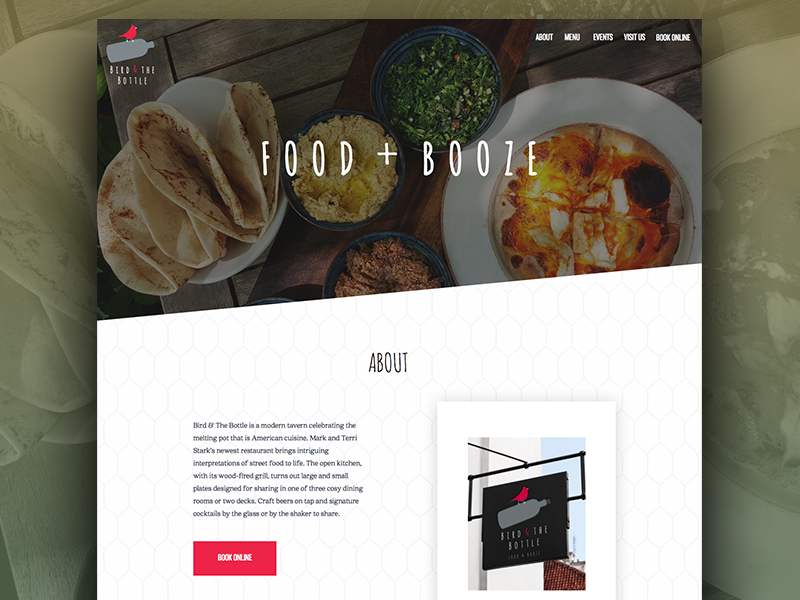### Advertisement for "Bed and the Bottle"

In the top right corner of the advertisement, the name of the store, "Bed and the Bottle," is prominently displayed. The imagery includes a grey bottle laid horizontally with a red bed positioned on top of it, visually reinforcing the store's name. The menus, written in white text, are also located in the top right corner and list the options: About, Menu, Event, Visit Us, and Book Online.

Centrally placed in white text is the bold statement "Food + Booze," drawing immediate attention. The background of the advertisement showcases an array of plated foods, featuring green vegetables, various doughs, and an assortment of other culinary delights, giving a vibrant and appetizing visual.

The bottom half of the advertisement features a white background with a black mesh pattern consisting of interconnected octagon shapes. In this section, there's a detailed "About" description that reads: 
"Bed and the Bottle is a medium tavern celebrating the melting point that is American cuisine. Mark and Terry Stark's newest restaurant brings intriguing interpretations of street food to life. The open kitchen with its wood-fired grill turns out large and small plates designed for sharing in one of three cozy dining rooms and two decks. Craft beers are available on tap, along with signature cocktails served by the glass or by the shaker."

At the very bottom, a red button invites viewers to "Book Online." To the right side of this section, there's an outdoor sign displaying "Bed and Bottle" in black text.